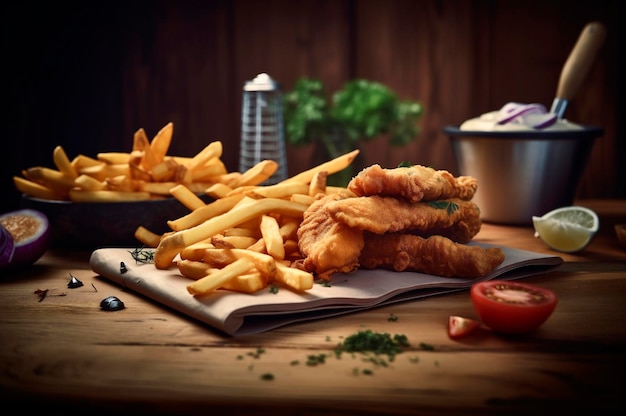The image captures a professionally taken photograph of freshly prepared food, featuring prominently in the foreground, a black bowl filled with French fries. To the left of the bowl lies an onion cut open, revealing its inner layers. Adjacent to it, there are French fries laid out on a napkin-covered surface, accompanied by what appears to be chicken tenders, although there's a possibility they could be fish, suggesting a fish and chips dish. Among the array of garnishes, a tomato slice and a lime or lemon wedge are visible, alongside a sprinkling of chopped parsley. The scene is set against a backdrop that is blurred but hints at wooden walls, interspersed with green plants, creating a cozy and inviting atmosphere. Additional elements include a small metal object and a container of dressing, topped with onion pieces, adding to the rustic and appetizing presentation.